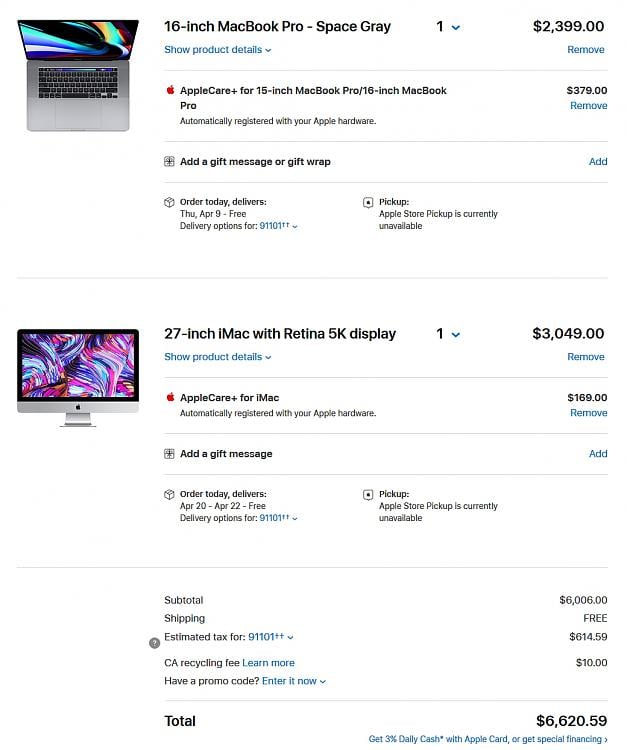Screenshot of an e-commerce website featuring MacBooks and Mac-related items. 

**First Item:**
- **Product:** 16-inch MacBook Pro in Space Gray
- **Price:** $2,399
- **Description:** The MacBook Pro is presented with a sleek, gray frame and features a dynamic wallpaper with swirling hues of blue, green, and red.
- **Add-ons:** AppleCare option available for $379.
- **Delivery Details:** Order today for free delivery by Thursday, April 9th. Pickup is unavailable.

**Second Item:**
- **Product:** 27-inch iMac with Retina 5K Display
- **Price:** $3,049
- **Add-ons:** AppleCare Plus for iMac available for $169.

**Order Summary:**
- **Subtotal:** $6,006 for both items.
- **Shipping:** Free
- **Estimated Tax for ZIP Code 91101:** $614.59 (including a $10 CA recycling fee).
- **Total Amount:** $6,620.59

**Additional Information:** Small blue text below the total amount indicates options for financial benefits: "Get 3% daily cash with Apple Card or get special financing."